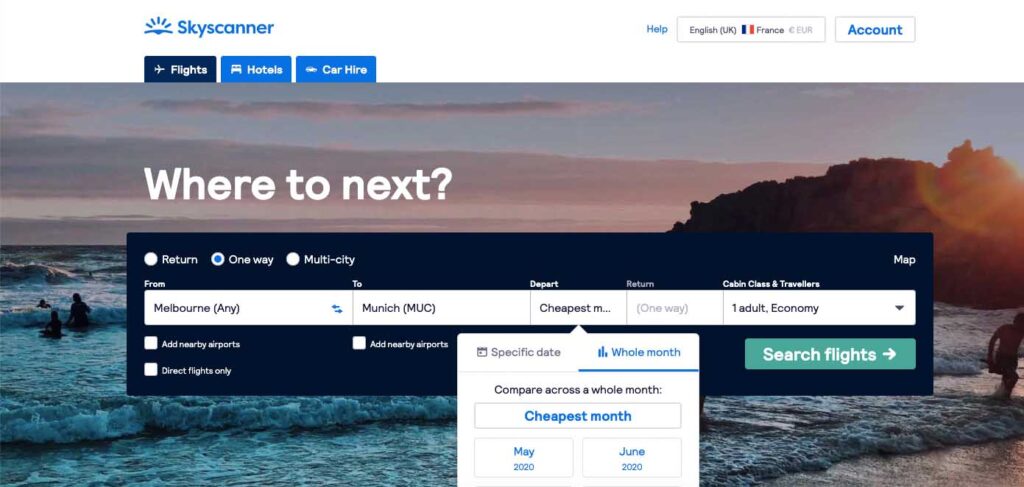Screenshot of a travel booking website, possibly a third-party service, with a navigation bar at the top left displaying "Sky Scanner" in blue alongside options for "Flights," "Hotels," and "Car Hire." The "Flights" tab is currently selected, with a prominent label stating "Where to next?" in white. The interface below includes fields for users to input their departure city, destination, travel dates, and seating preferences.